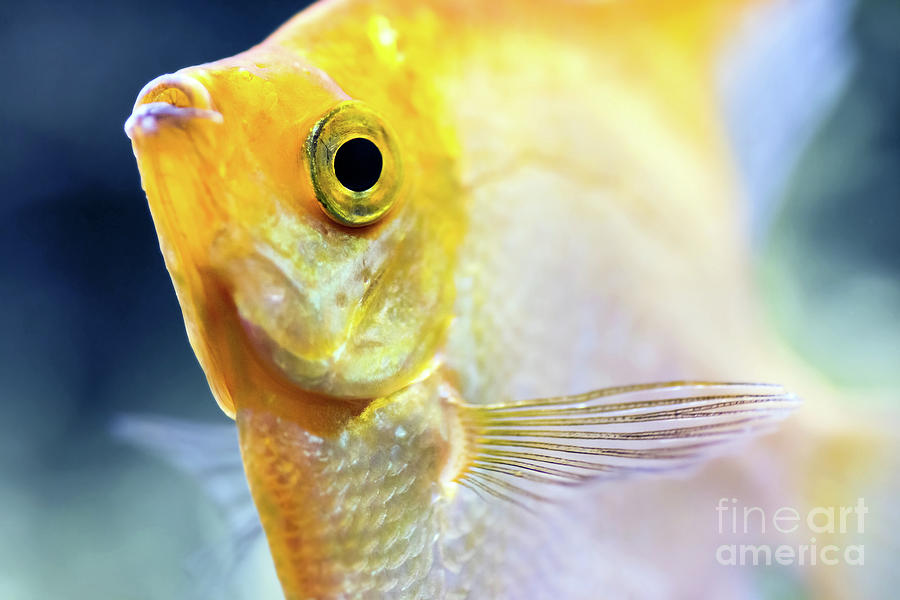This close-up photograph captures the striking face of a goldfish swimming underwater. The goldfish, with its bright and brilliant yellow head, is in sharp focus while the rest of its body and surroundings are blurred. The fish is oriented to the left, revealing one large, round black eye and slightly open mouth. The fine details of the gills beneath its head exhibit an iridescent, silvery-white hue. The translucent fin near its head is partially visible, with yellowish spines adding to the intricate texture. The background features a gradient of blue and green, enhancing the underwater effect. In the bottom right corner, there is a translucent watermark that reads "Fine Art America." The composition emphasizes the vivid colors and detailed features of the goldfish, especially its vibrant yellow head and deep black eye, set against the serene aquatic backdrop.